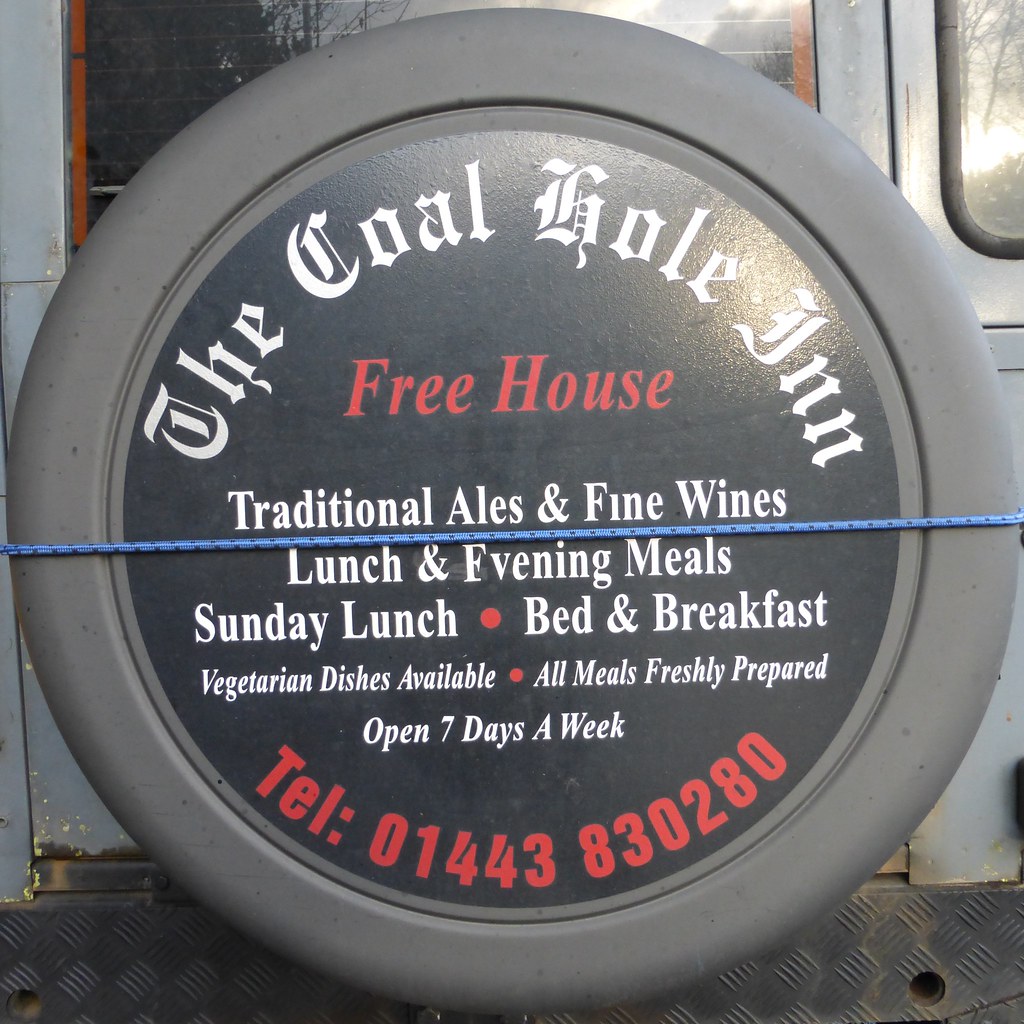The image is a photograph of the back of a gray vehicle featuring an advertisement attached to a circular spare tire holder. This circular object is a back wheel adorned with a large black sticker bearing white and red text. At the top center of the circle, in white Old English font, it reads "The Go Whole Inn." Below this, in red letters, it states "Free House." Further down, a list in white letters describes the offerings: "Traditional Ales and Fine Wines," "Lunch and Evening Meals," "Sunday Lunch," "Bed and Breakfast," "Vegetarian Dishes Available," "All Meals Freshly Prepared," and "Open Seven Days a Week." At the bottom, the telephone number "01-443-830-280" is prominently displayed in red. In the background, the gray vehicle features two windows at the top right with a reflection of a tree, and a metal bumper is visible at the lower part of the image. Additionally, a blue rope is tied around the wheel, securing it in place.